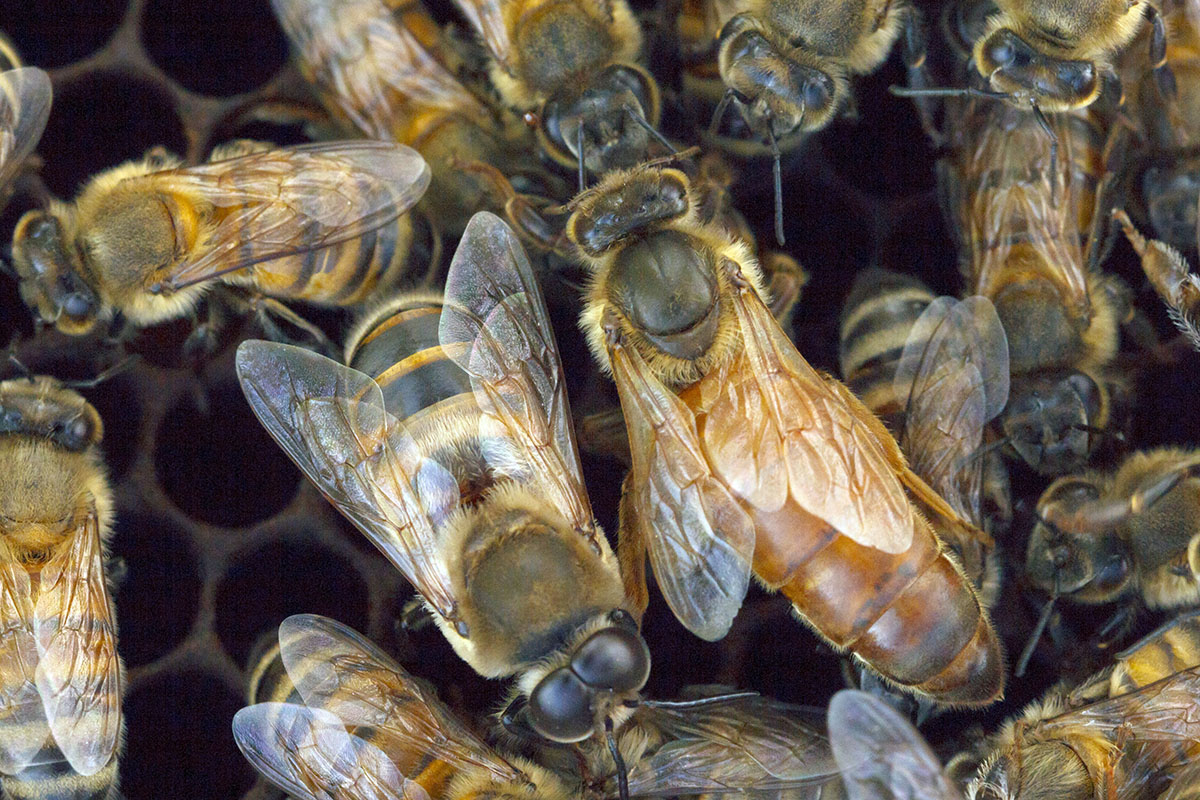In this detailed close-up image, we see a vibrant and bustling beehive. The background is filled with dark brown honeycombs composed of hexagonal cells, immediately signaling the hive setting. In the center of the image, two prominent bees take focus, their delicate, transparent wings shimmering as they orient their bodies in different directions—one looking towards the bottom and the other towards the top of the frame. Around them, at least a dozen bees are visible, with bodies displaying a beautiful mix of golden, black, reddish, and yellow hues adorned with black stripes. Large black eyes and antennae add to their distinct features. The bees' bodies are partially covered in fur, especially around their heads, and their legs and wings jut out in various postures, suggesting constant movement. Amongst this crowd, a larger bee, possibly the queen, stands out with its more yellow coloration. The bees crawl over each other and group together closely, emphasizing the hive’s dense and active environment.